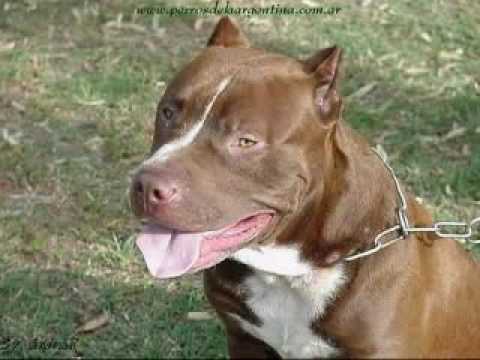This image depicts a brown and white pit bull with a slightly shiny chocolate-colored coat. The dog's head, neck, and shoulders are prominently displayed, with its body sloping downward, suggesting it is sitting in a grassy area that appears worn and patchy. The background features green grass with some brownish-gray patches, as well as scattered leaves indicating it is a daytime outdoor setting. 

The pit bull has a distinctive white stripe that runs down from the middle of its forehead to its nose and a white patch on its chest. The dog's short, pointy ears and open mouth with the tongue slightly protruding give it a neutral expression, neither happy nor sad. The photo captures the dog glancing sideways, providing a partial profile view that shows both of its eyes.

Around the dog's neck is a silver chain, which functions as a choke collar extending out of the frame, emphasizing the restrained nature of its position. Text at the top of the image includes a partially legible URL, possibly indicating a website related to purebred dogs.